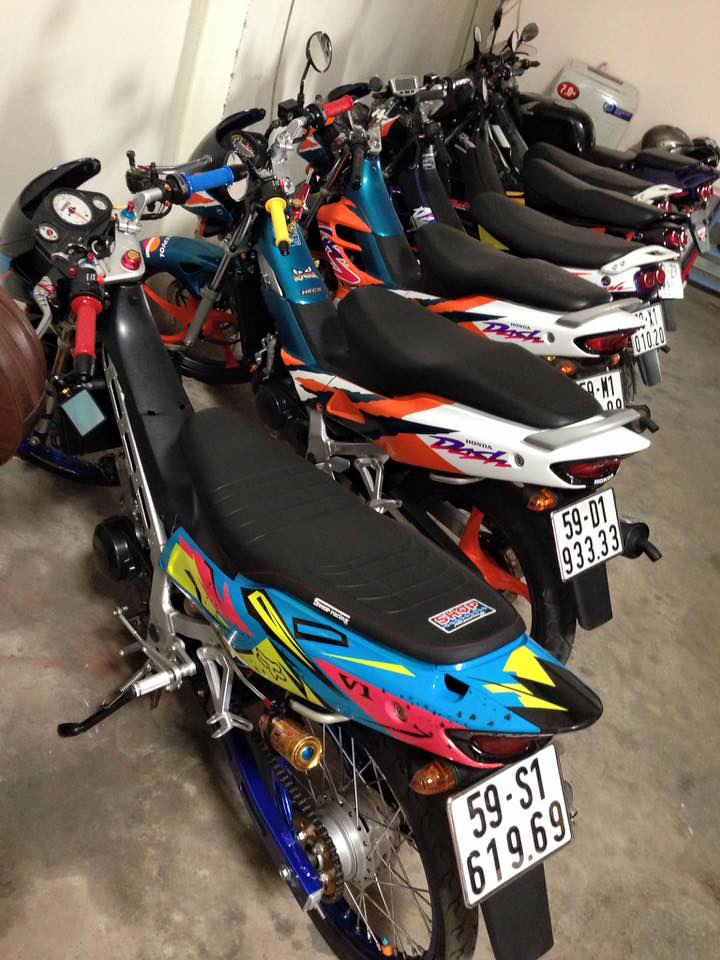The image features an indoor setting with a white or off-white wall and a cream-colored far wall. The ground appears to be a concrete surface. The scene is dominated by a lineup of seven brightly colored motorcycles, possibly dirt bikes or mopeds, parked in a neat row facing approximately the 10 o'clock position. The motorcycles display a variety of vibrant colors, including blue, red, white, and combinations thereof. Each bike is equipped with a black seat and various colored handlebars. The front motorcycle stands out with a long black seat, painted blue with additional yellow and pink accents. All motorcycles feature unique license plates with a format not typical to American styles, including combinations of letters and numbers like "59S1" or "V1," and detailed as "59S1619.69" on one of them. Several bikes also display the Honda brand. Behind the motorcycles, a gray metal object is visible, adding to the industrial indoor ambiance.